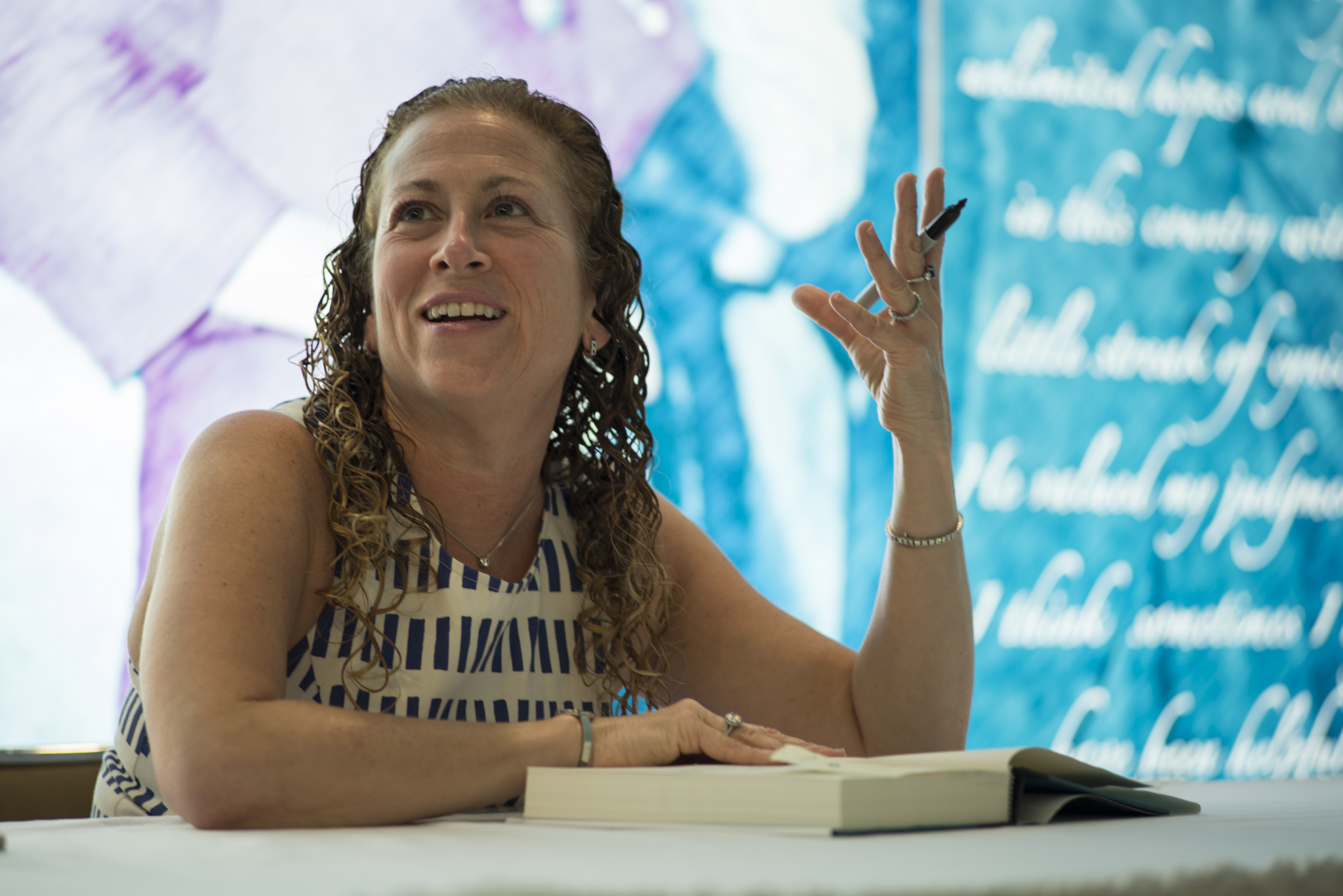In this image, a woman with long, curly hair that cascades in shades of brown, pink, and blonde sits at a white table with a thick, open book in front of her. She is smiling and looking to her right. Her curly hair reaches down to her chest, and she wears a distinctive sleeveless top featuring a white and dark blue thatch design. On her left wrist, she wears a bracelet, and her left hand is adorned with several rings. Additionally, her left hand holds a black Sharpie marker. On her right wrist, she wears another bracelet and a diamond ring. The backdrop behind her consists of blurred cursive writing, set against a blend of blue, purple, and pink hues, suggesting it might be part of a presentation setup.